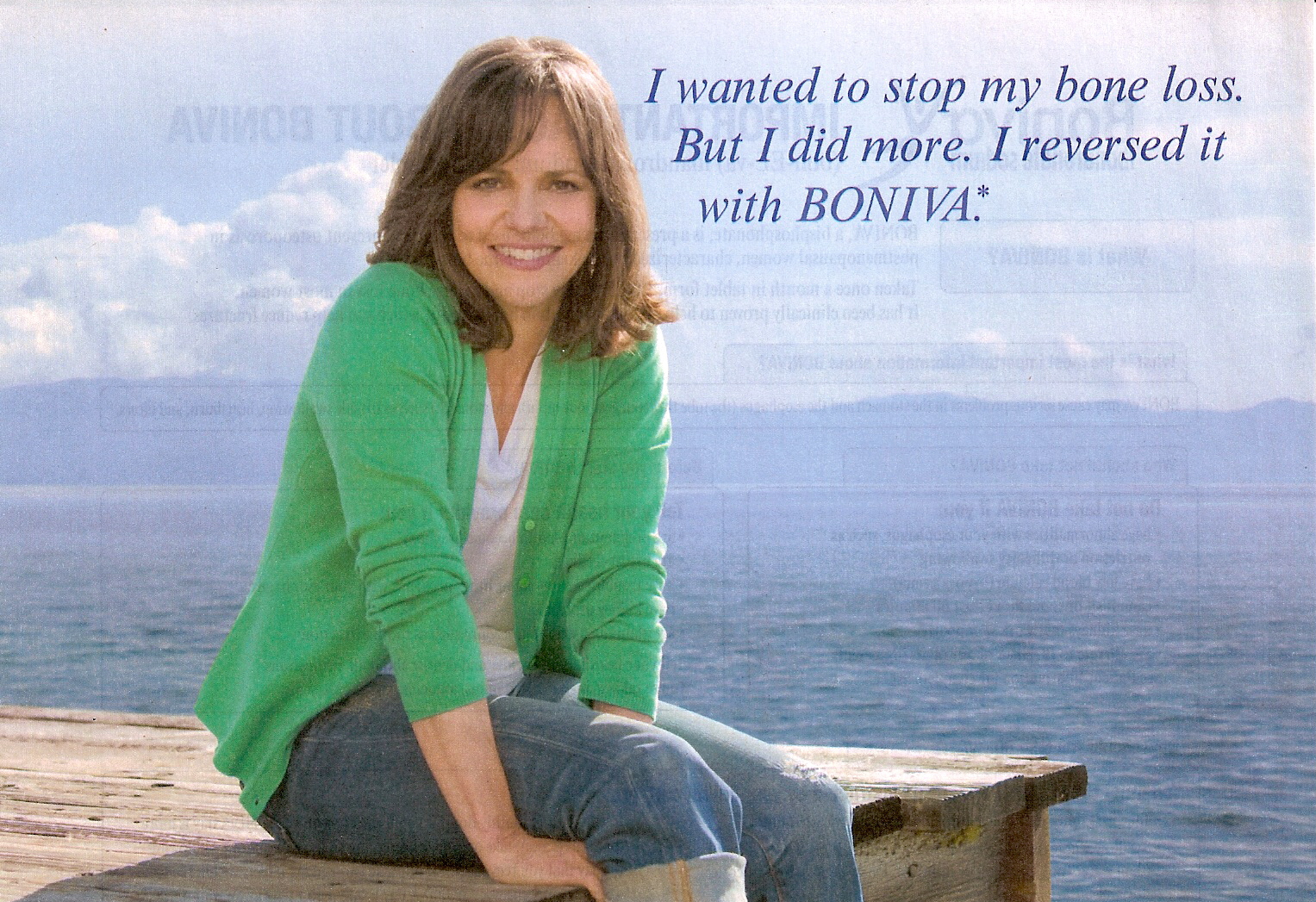In this image, a woman sits on the edge of a brown wooden dock that extends into a vast, calm blue body of water, which could be an ocean or a large lake. In the background, there is a mountain range peeking through the left-hand side, partially covered by a scattered cluster of clouds, under a bright blue sky. The woman, who bears a resemblance to a young Sally Field, is smiling and looking towards the camera. 

She is dressed casually in a green sweater that is open, revealing a white V-neck shirt underneath, and blue jeans rolled up to knee length. Her right leg, from the knee down, suggests she is possibly wearing a boot. Her brown hair falls to around her shoulder level. At the upper right corner of the image, the text “I wanted to stop my bone loss. But I did more than that; I reversed it with Boniva.” is prominently displayed in red and blue font.